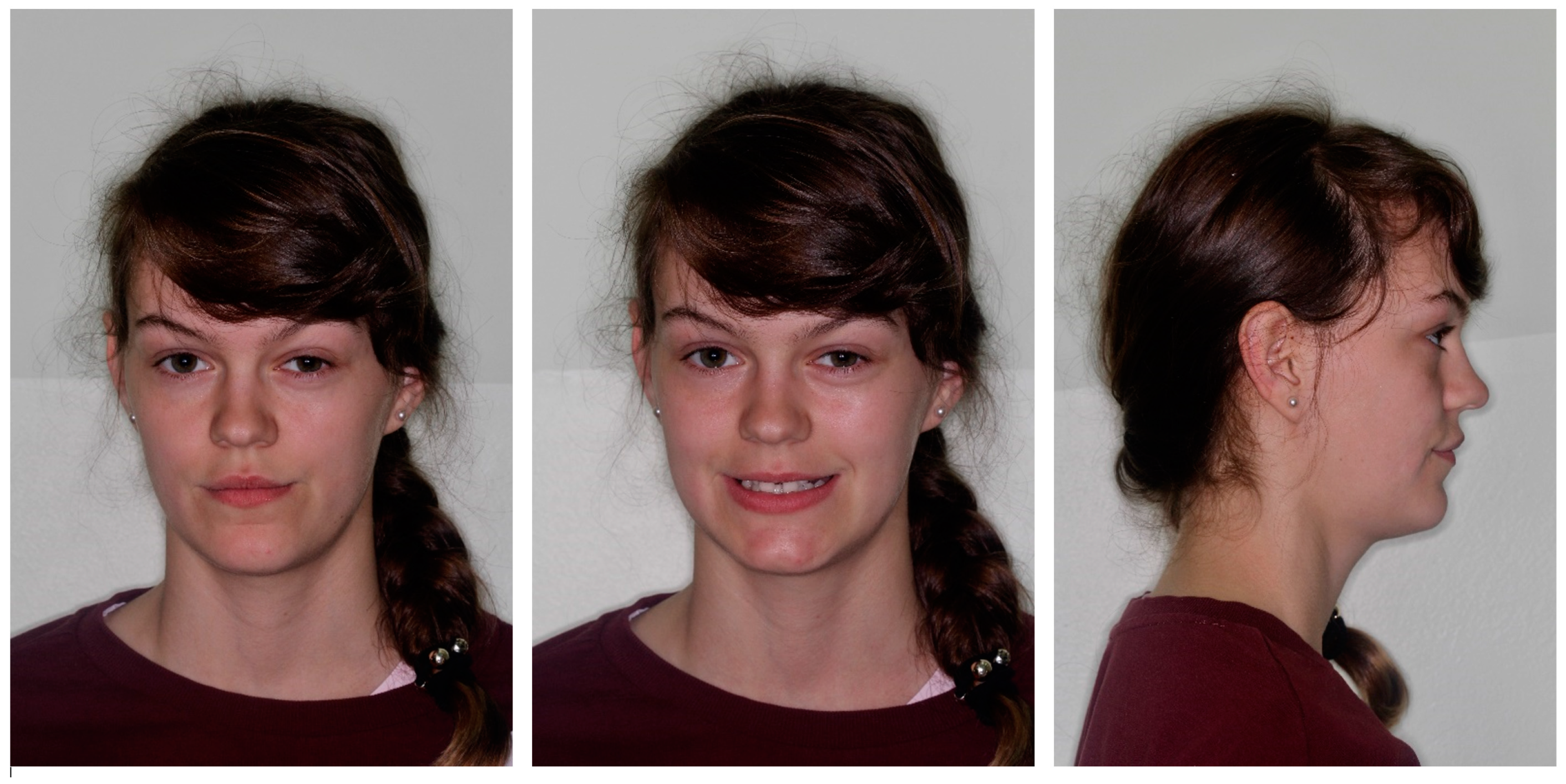This tri-panel photograph captures a young woman, possibly a teenager, in three distinct poses. Each panel is a headshot of the same person with varying expressions. In the first image on the left, she faces the camera straight on with a neutral expression, her chestnut-colored hair styled with bangs sweeping over her left eye, and a ponytail falling over her left shoulder. She's dressed in a maroon or dark red shirt layered over a white shirt. She has earrings and possibly a hair clip.

The second image in the middle mirrors the first in position and framing, but this time she has a slight smile, adding a touch of warmth to her expression.

The third image on the right presents a right-side profile view. Her hair reveals some loose strands hanging over her right forehead and cheek, with her ponytail still visible over her left shoulder. She gazes to the left with a smirk on her face, her expression hinting at indifference or nonchalance. Her eyes and pink lips stand out, while her attire and accessories remain consistent across all three photos. This detailed arrangement allows for a comprehensive view of her varied expressions and nuanced appearances.